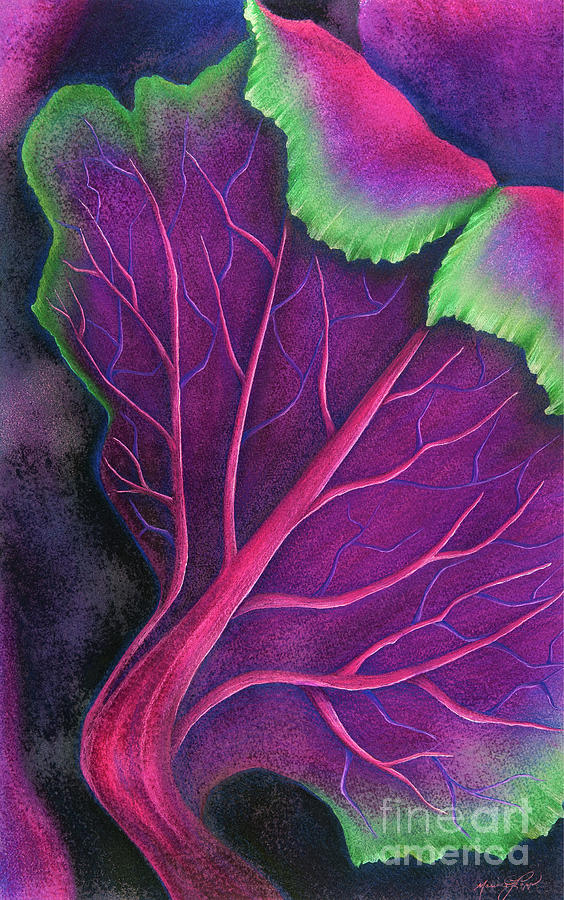This abstract, botanical art piece, possibly a digital creation resembling a painting, depicts a close-up of the underside of a large, notably intricate leaf, like rhubarb or potentially cabbage. The artwork, presented in portrait mode, is approximately twice as tall as it is wide. Its dominant focus is a network of elaborate veins and roots, which start from a central stalk and branch outwards in a tree-like structure. These veins are vividly colored, intermingling shades of blood red, dark purple, lighter pink, and some blue, mimicking the appearance of arteries and veins. The leaf itself exhibits a gradient of colors, beginning with green edges that transition into purple, then dark red, and finally lighter red hues. The stalk ascends at a 45-degree angle from the center towards the left upper corner before it bends sharply towards the upper right corner, giving the leaf a drooping, three-dimensional effect. The image is detailed enough that one can observe the fine, textural nuances in the veins, resembling a mix between oil colors, crayons, or colored pencils. In the lower right corner, there is an overlay of semi-transparent gray text that reads "fine art america."